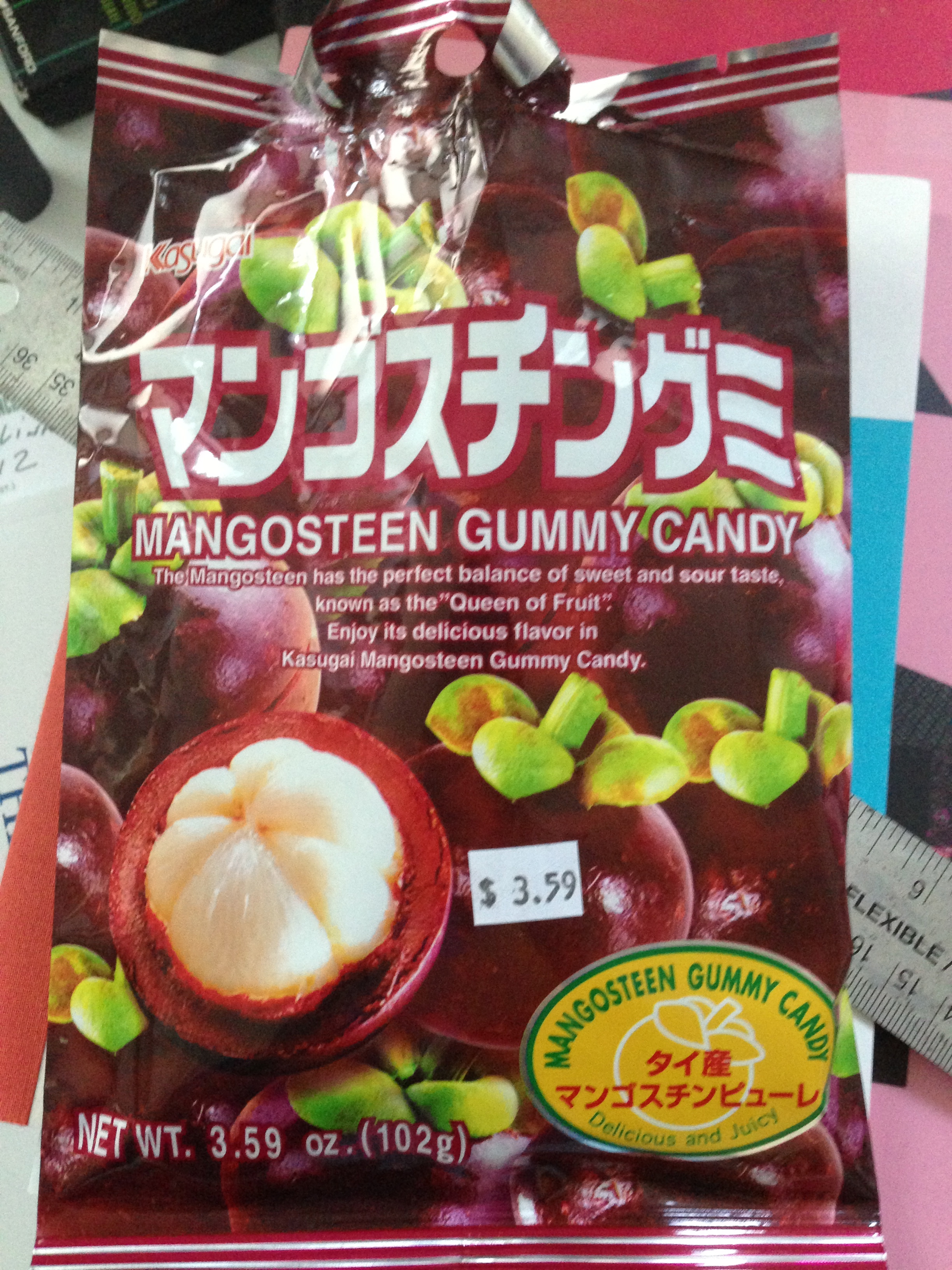The image depicts a package of Kasugai Mangosteen Gummy Candy, prominently displayed on a cluttered desk. The packaging is predominantly deep red with green leaves and variously colored fruits scattered throughout, primarily showcasing mangosteens, which are green and orange, resembling plums. Central to the design is text in Japanese, with the English translation "Mangosteen Gummy Candy" immediately below, rendered in white with a red outline. A descriptive passage informs that the mangosteen, known as the "queen of fruit," offers a perfect balance of sweet and sour flavors. Additional details, such as "NET WT 3.59 ounces (102 grams)" appear in the bottom left corner, with a yellow circular label on the right stating "Mangosteen Gummy Candy: Delicious and Juicy." The price tag, $3.59, is affixed centrally on the package. In the background, a ruler marked "flexible" displays measurements, and various indistinct papers and a box labeled "Banford" are visible, but the main focus remains the vibrant candy package.